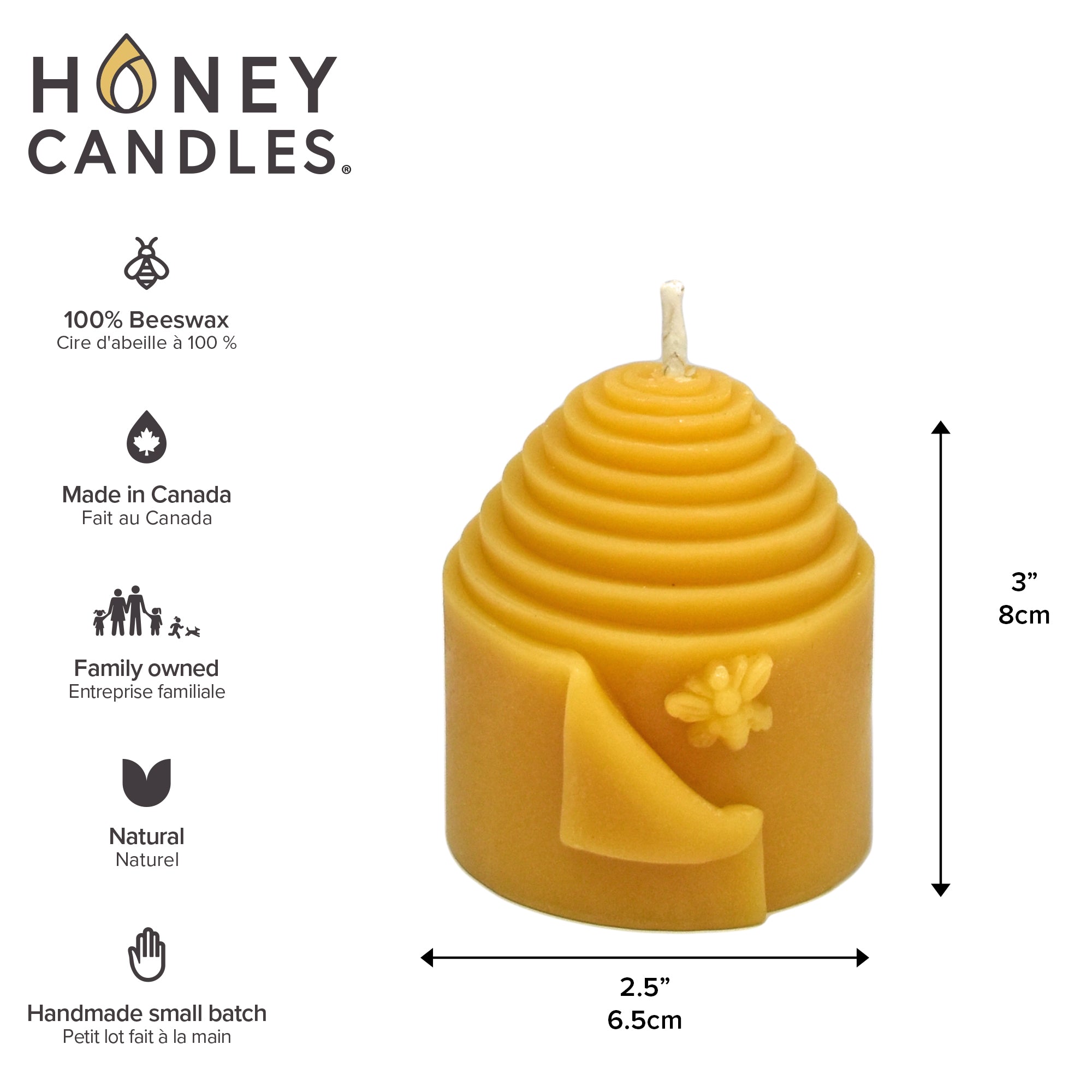This image is a detailed product photo of a honey-colored beeswax candle, featuring a terraced design that resembles ribbons wrapped around each other, culminating at the top where a white wick protrudes. The base of the candle is wider and slightly folded back to reveal a small bee imprint. To the right of the candle, dimension markers indicate its size as 3 inches (8 centimeters) in height and 2.5 inches (6.5 centimeters) in width.

In the upper left corner, the logo "Honey Candles" is prominent, with the 'O' depicted as an orange flame. Below the logo, a series of bullet points with corresponding icons provide additional details: a bee icon denoting 100% beeswax, a water droplet with a Canadian maple leaf signifying Made in Canada, a stick figure family representing Family Owned, a tulip symbolizing Natural, and a hand icon indicating Handmade Small Batch. Each bullet point is clearly labeled and contributes to the artisanal presentation of the candle.